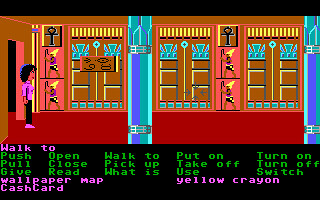The image captures a scene from what appears to be a vintage video game. The setting is a large open room adorned with a plush red carpet that extends across the floor, providing a striking contrast to the room's prominent turquoise blue columns that stretch from the carpet to the ceiling. The walls are clad in brown paneling, giving the space a warm, retro ambiance. On the far left side of the room, an open doorway reveals the presence of a young boy standing just inside the entrance. He is dressed in a white shirt, black pants, and white tennis shoes, and his posture suggests he is ready for adventure within this digital world. At the bottom of the image, a black interface panel displays green and purple pixelated text, listing various commands such as "walk to," "push," "open," "pull," "close," "give," "read," "pick up," "put on," and "take off," indicating the interactive elements typical of classic point-and-click adventure games.